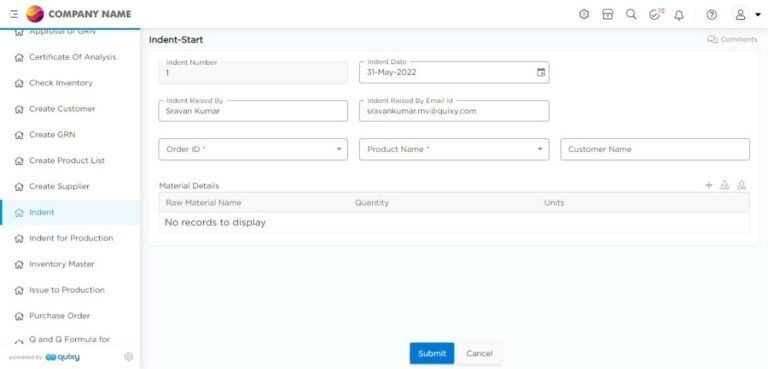This is a detailed screenshot of a website template designed for a company. The template appears to be a comprehensive tool for various business operations. At the top, it prominently displays "Company Name." The interface includes numerous functionalities such as:

- **Approval of GRN**
- **Certificate of Analysis**
- **Check Inventory**
- **Create Customer**
- **Create GRN**
- **Create Product List**
- **Create Supplier**
- **Indent Management:** Allows users to manage orders with fields for Indent Number, Indent Date, Indent Raised By, Indent Raised By Email ID, Order ID, Product Name, Customer Name, and Material Details.
- **Inventory Master**
- **Issue to Production**
- **Purchase Order**
- **Q&Q Formula**

Currently, the page is on the "Indent Start" section where users can enter details such as indent number, indent date, indent raised by, and other relevant information. The material details section currently displays "No records to display," indicating that this is where users would add pertinent details.

At the bottom of the page, there are two buttons: a blue "Submit" button with white text, and a white "Cancel" button with black text.

This template appears to be a versatile tool for customizing and managing various aspects of a company’s operations, including production numbers, products, and customer data. It provides a personalized approach to managing business processes, recognizing that each company has unique needs.